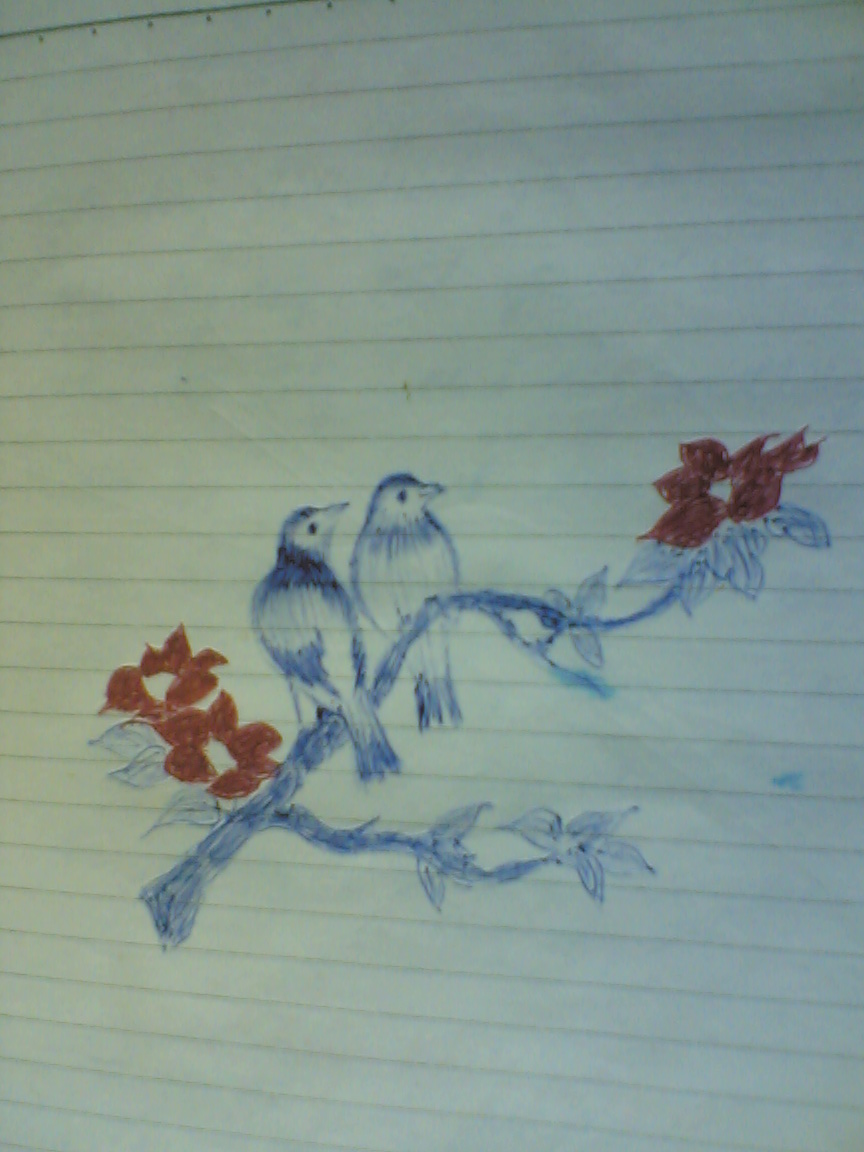This is a detailed pen and ink drawing on lined notebook paper, executed primarily in blue and red ballpoint pen. The artwork has the feel of an Asian painting due to its elegant composition and subject matter. Central to the image is a gracefully curving branch adorned with leaves and vibrant red flowers that resemble poinsettias. Perched on this branch are two small birds. The first bird, positioned to the left, faces away from the viewer yet has its head turned to the right, looking toward the flowers. The second bird, situated to the right, faces the viewer, revealing its belly and tiny feet as it, too, turns its head toward the red blooms. Below the birds, another twig diverges from the main branch, sprouting additional leaves and a cluster of two more red flowers to the left. The overall effect is delicate and serene, capturing the tranquil beauty of nature with a minimalist yet detailed aesthetic.